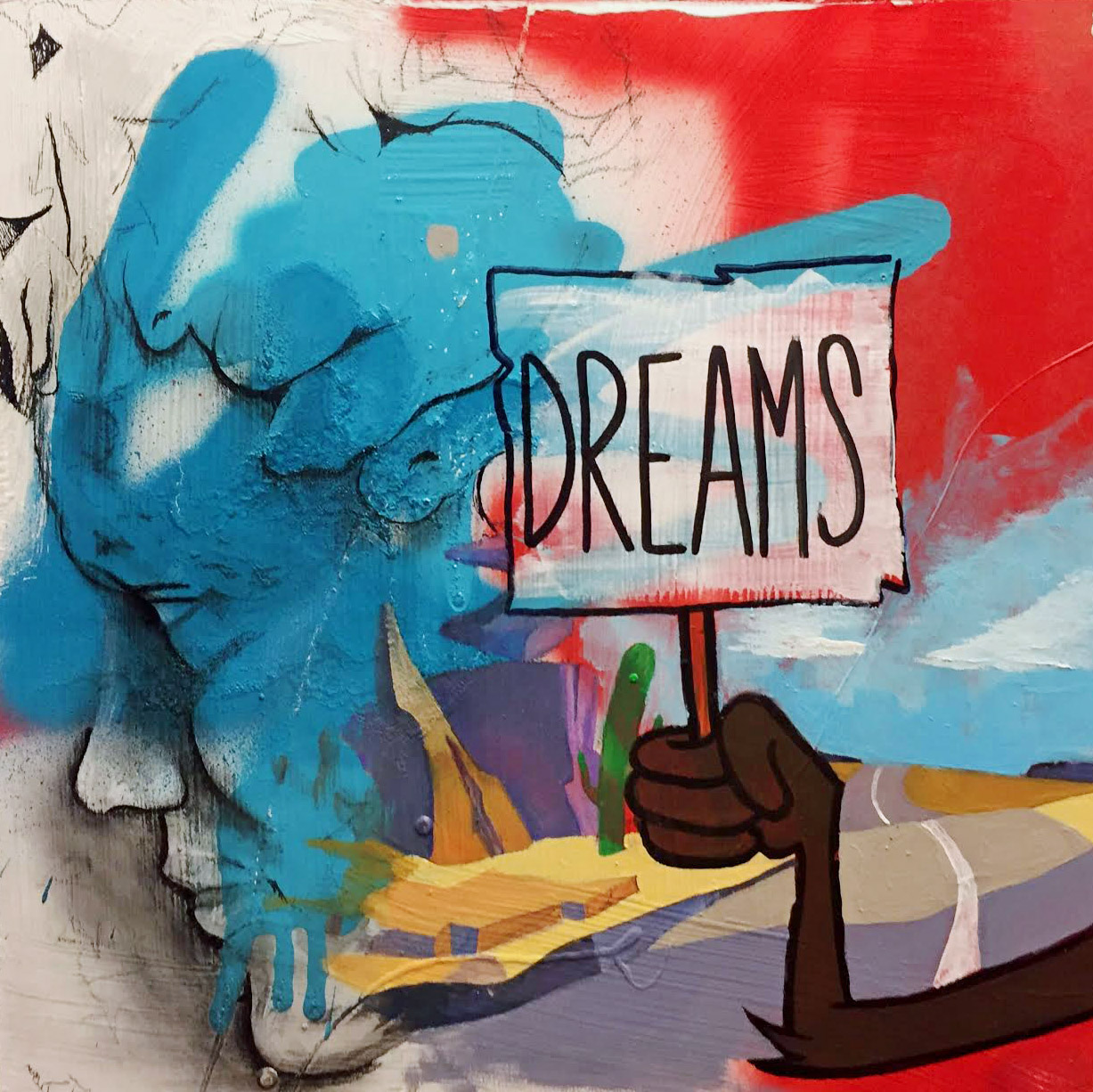The image is a vibrant, multi-colored piece of graffiti art on a white wall. Dominating the center is a brown, anthropomorphic arm, reminiscent of Wile E. Coyote's from Warner Brothers' Looney Tunes, holding a bold sign that reads "DREAMS" in black capital letters. The arm extends vertically from the right side of the image.

To the left, there's a detailed side profile of a person's face, looking leftward. The face, possibly representing a young Black individual, is primarily white with areas covered in blue paint, giving it a unique and layered appearance. This blue paint extends to the hair, creating a striking visual contrast. 

The background features a desert-like scene with a road running through the middle, characterized by a white line dividing the lanes. A purple-shaded mountain and a tall green cactus are visible on the left side, accentuating the arid landscape. Above, the sky is blue, dotted with white clouds, adding depth to the composition. Additionally, the top right corner of the image is filled with red paint, further contributing to the graffiti's colorful and chaotic nature.